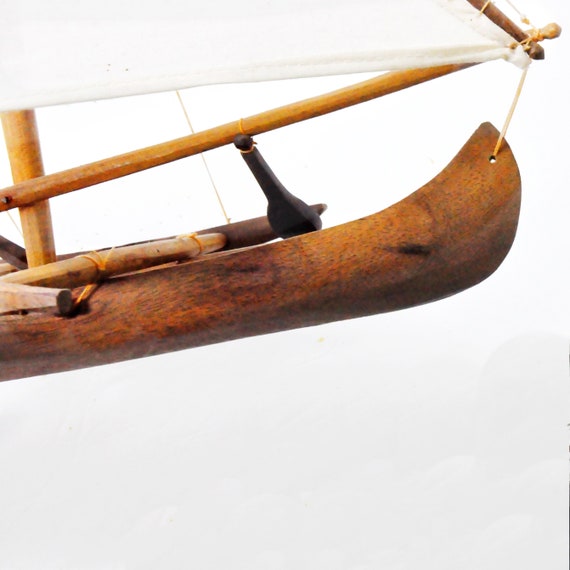The image is a detailed close-up of a handcrafted wooden model boat. The boat, visible primarily in the upper portion of the square, white-backgrounded photo, showcases its brown wooden construction, emphasizing the back part of the vessel. The craftsmanship includes wooden rods extending from the base, which support a pristine white sail. Several ropes elegantly connect the sail to various parts of the boat, accentuating the model's intricate design. This small, artistic representation of a boat appears finely built, potentially serving as a decorative piece. The zoomed-in focus provides an intimate look at the boat's elegance without revealing its entirety, sitting against a light gray, almost white backdrop.